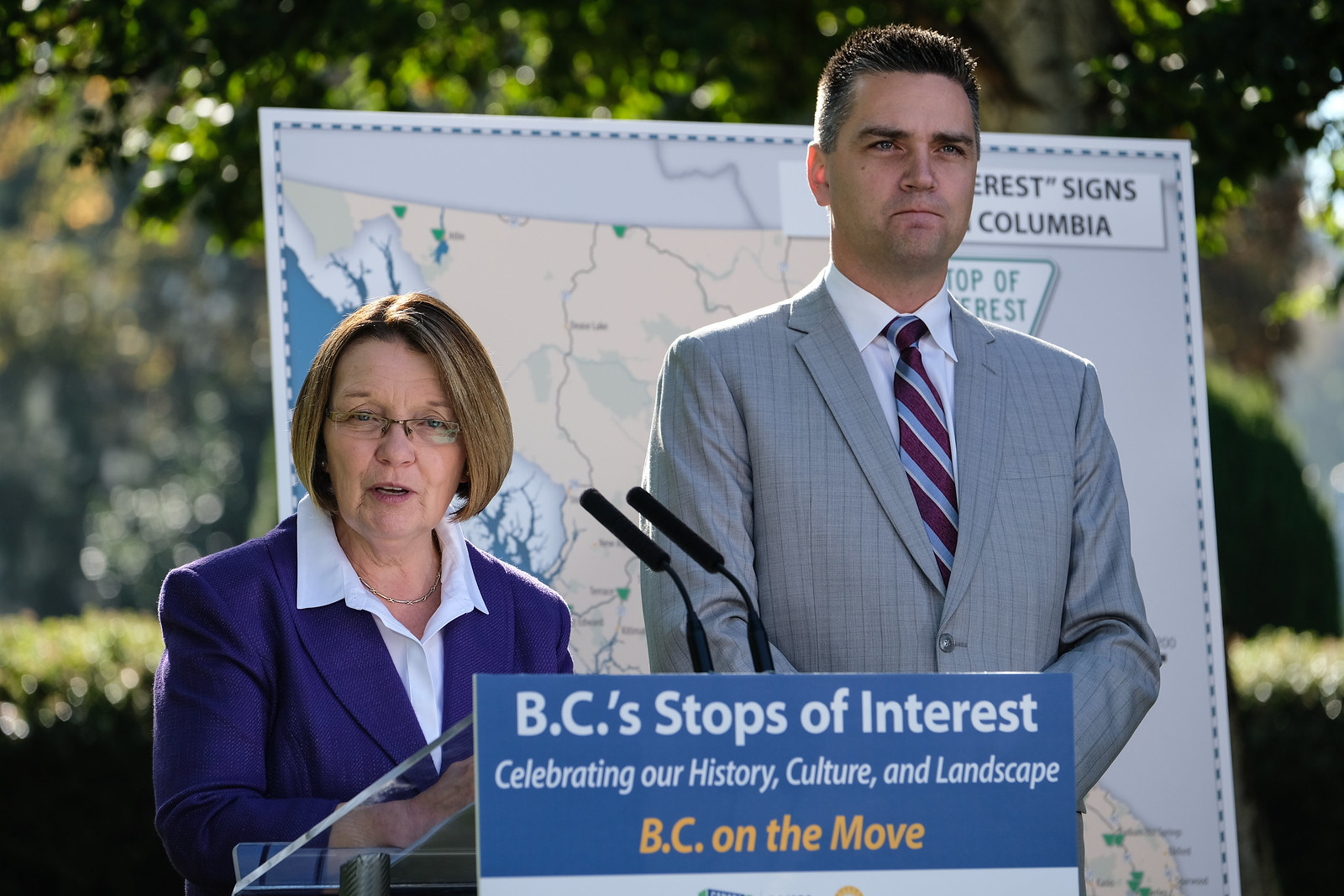In this detailed photograph, a man and a woman are standing side by side outdoors, behind a transparent glass podium equipped with two black microphones. The scene appears to be set for a speech or announcement. The woman, who is speaking into the microphones, is positioned on the left. She is wearing a white collared shirt and a blue coat, complemented by a silver necklace and wire-rimmed glasses. She has light skin and shoulder-length medium brown hair. To her right stands a man wearing a light grey checked suit, paired with a white collared shirt and a maroon and grey striped tie. He has medium skin and black hair, and he is looking straight ahead with a neutral expression, his lips slightly parted.

On the front of the podium is a blue sign with white text that reads, "BC's Stop of Interest." Below this, in smaller white letters, it reads, "Celebrating our history, culture, and landscape," and at the bottom, in yellow letters, is "BC on the Move." Behind the speakers, a large map is displayed, partially obscured by their presence. Further in the background, blurred images of trees and bushes can be seen, adding to the outdoor atmosphere. The combination of these elements paints a vivid picture of a formal event, likely celebrating or announcing something significant related to British Columbia’s heritage.